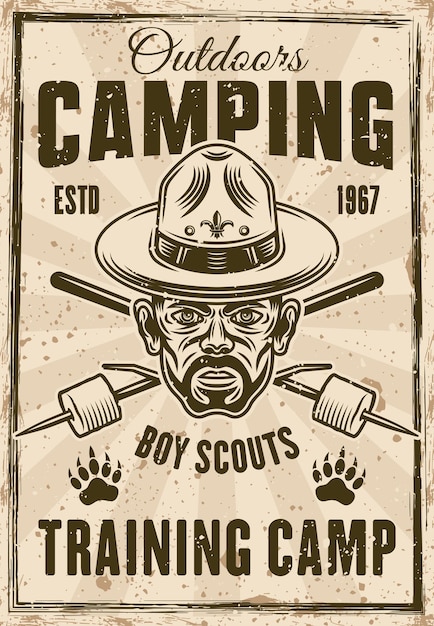The image depicts a vintage-style metal decor sign with a tan background and a dark brownish-black border. The sign prominently features the text "Outdoors Camping Established 1967 Boy Scouts Training Camp." At the center of the design, there is a detailed illustration of an older man with a beard, goatee, and a Boy Scout leader's hat. His expression appears stern or scowling. Above the phrase "Training Camp," two bear paw prints are visible. Overlaying the man’s image are two crossed sticks, each with a marshmallow on it, reminiscent of a campfire setting. The text is a mix of cursive and block lettering, adding to the rustic aesthetic of the piece. This sign would be an ideal decorative item for an outdoor-themed space.